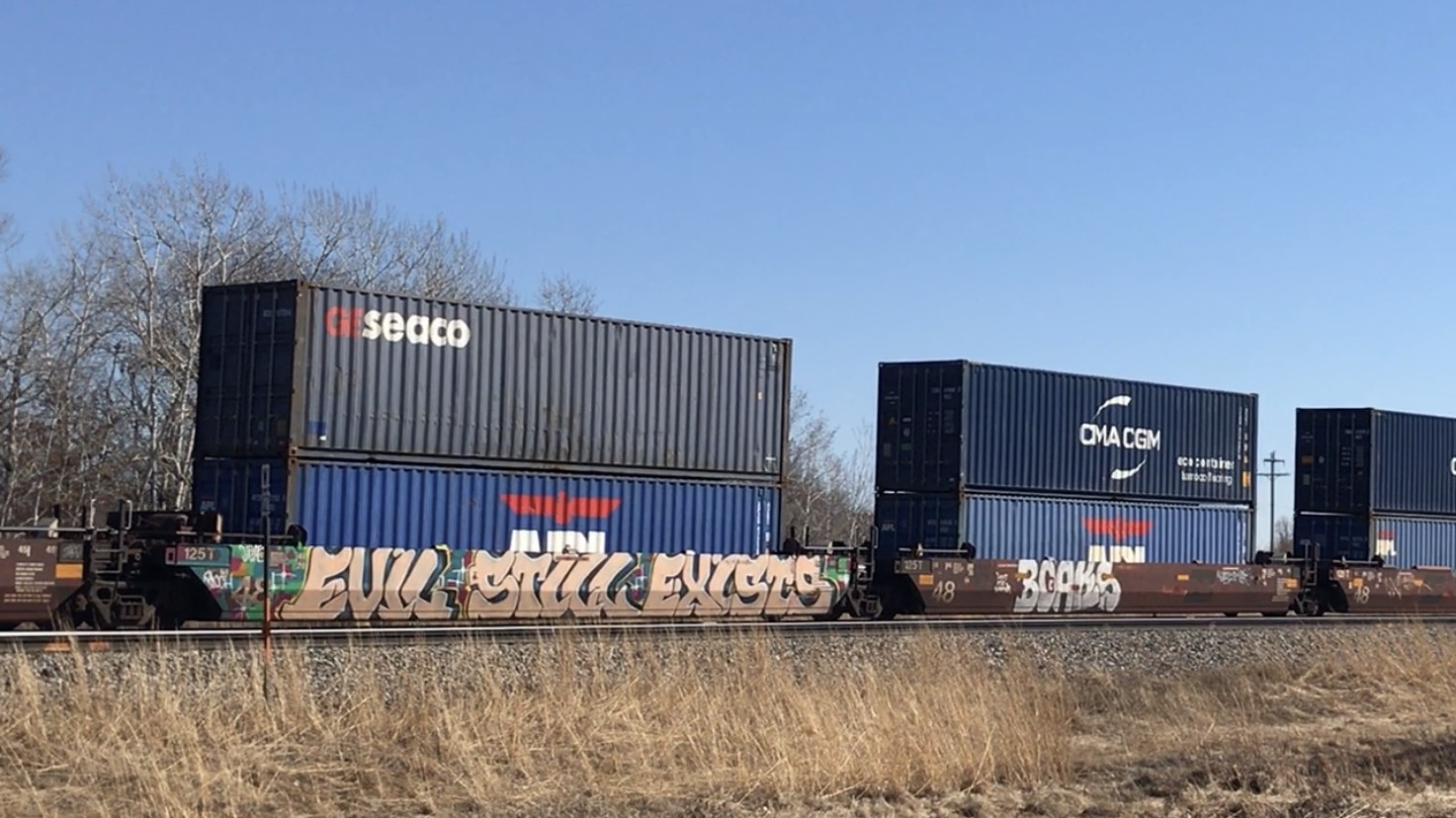In this vibrant, daytime outdoor photograph, a crisp blue sky, devoid of clouds, sets the scene. Bare trees and brownish-yellow dried grass surround the area, indicating it was taken in late fall or early spring. Centrally positioned is a freight train with shipping containers stacked two by two along several railway carts. The train tracks, with their silvery gleam, cut through the center of the image, bordered by rocky ballast. Each container bears its own unique marks: the dark blue top containers read "Seaco" while the light blue bottom ones read "CMA CGM." Notably, two of the containers are adorned with graffiti—one in bold bubble letters proclaiming “Evil Still Exists.” Behind the train, a telephone pole stands symmetrically between the cars, contributing to the photo's structured composition, and a sparse arrangement of leafless trees rises in the background.